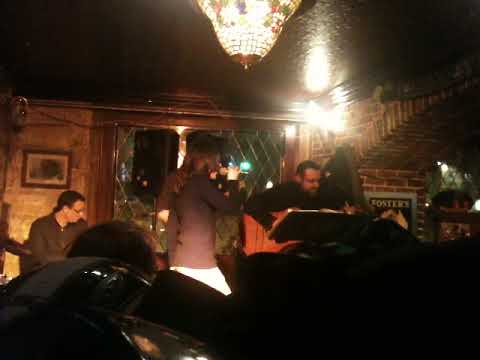The image depicts an indoor setting, likely inside a pub or bar, characterized by wooden woodwork and a brick archway on the right side. The scene is somewhat out of focus and overexposed, yet it clearly captures a musical performance in progress. Central to the image is a woman holding a microphone to her mouth, seemingly singing, while to her right, a man in a black shirt sits with an acoustic guitar on his lap, reading from sheet music. Behind them, another man appears to be seated, possibly engaged in playing a keyboard or drums, though details are obscured by the blur. To the left of the performers, two individuals stand facing the camera, though their roles are unclear. A notable element is a bright, ornate light fixture at the top center, casting a glare across the scene. The background features a mixture of wooden frames, glass, and a brick area with a sign bearing the word "Fosters." Darkness in the foreground adds an additional layer of obscurity to some items. The setting and scattered details suggest a lively, perhaps intimate musical event within a warmly decorated venue.